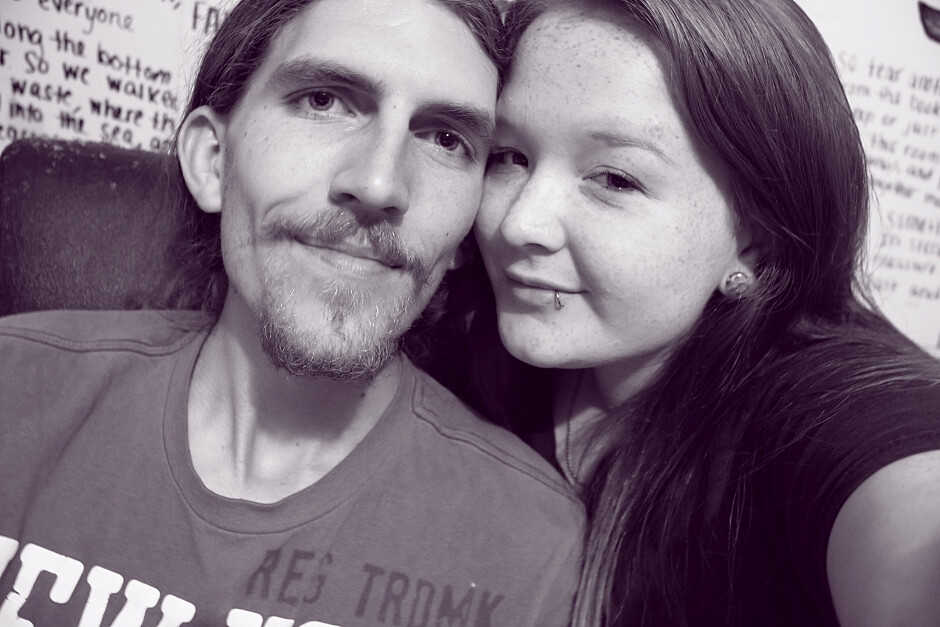This black and white photograph features a close-up of two individuals, a man and a woman, positioned at the center of the image, with their heads and upper shoulders prominently in view. The man on the left, who sports a goatee and dark hair, is looking directly at the camera with a slight smile. He is dressed in a dark t-shirt. The woman on the right has straight dark hair cascading down and is also wearing a dark t-shirt. She has a lip ring and her forehead and cheeks are touching the man's side. Both individuals are smiling subtly as they sit closely together in what appears to be a chair. The background is predominantly white, featuring some handwritten text on a poster board, though it is largely obscured by the subjects’ heads and thus unreadable. The setting appears to be indoors, possibly an educational environment, and no other objects are visible in the frame.